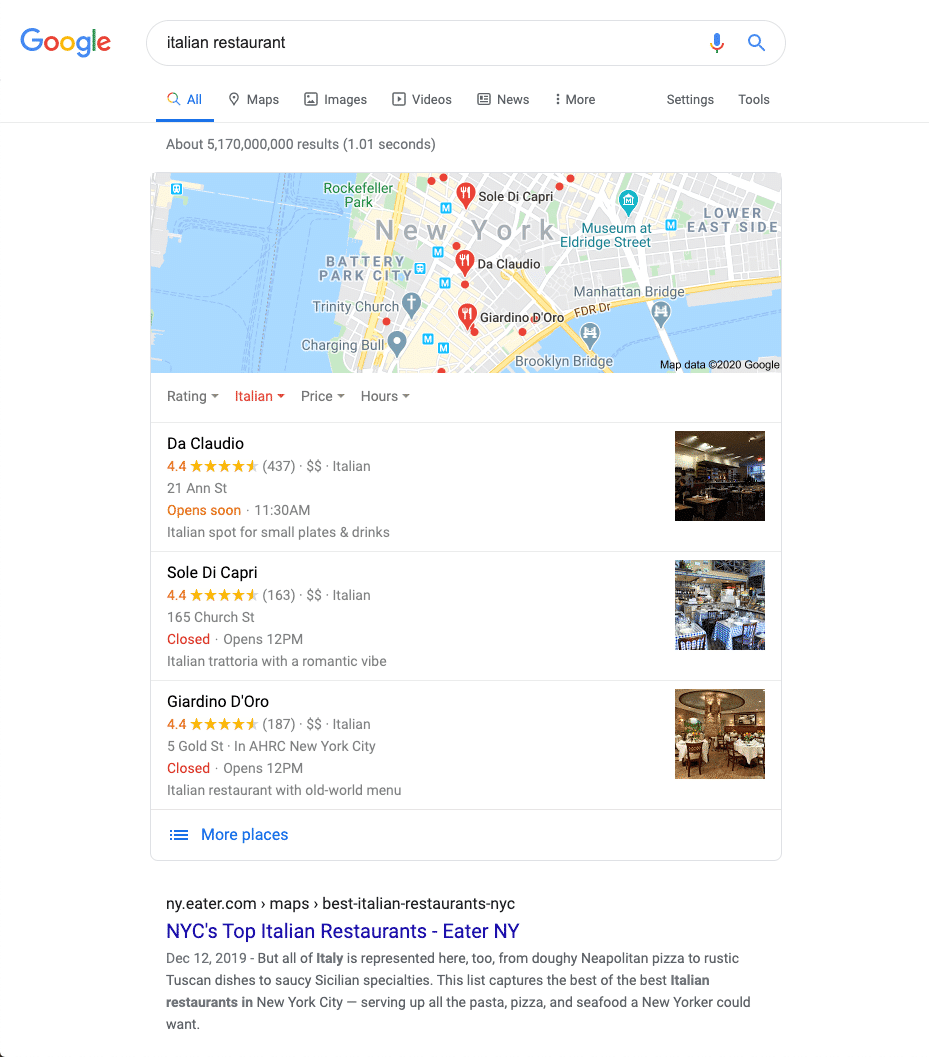This image, sourced from a Google search page, centers around a search query for "Italian restaurant." At the top, a search bar with the query "Italian restaurant" is clearly visible. Below the search bar, the interface displays a street map of New York City on the upper left side, providing geographical context. Beneath the map, three prominent Italian restaurants are listed: Di Claudio, Sol Del Capri, and Giardino D'Oro. Each restaurant entry includes a review rating of 4.4 out of 5 stars, accompanied by the address and current operational status (e.g., whether it is open or closed at the time). To the right of each restaurant's descriptive details, there are small, square photos showing the interiors of these dining establishments, offering a visual glimpse into the ambiance of each venue.